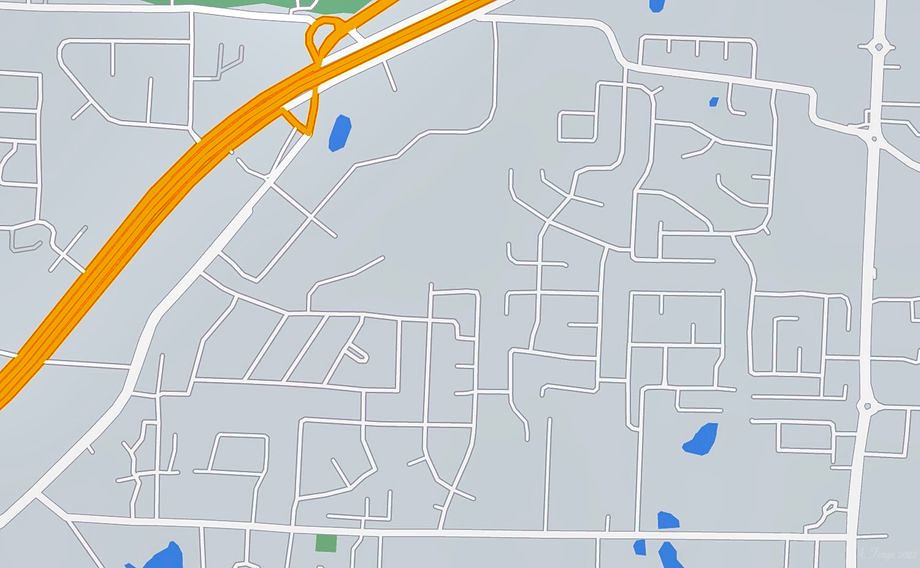The image depicts a simplistic, gray-scale representation of a city map, either a digital screenshot or an artistic drawing. The map features a network of white lines symbolizing various streets; some form closed shapes indicative of residential neighborhoods, while others are broader with intersections, suggesting more prominent thoroughfares. In the top left corner, a substantial orange line likely denotes an expressway or highway. Sporadically, small blue dots appear, presumably representing bodies of water. This map, however, is starkly minimalist, with no labels or detailed features, giving it an unfinished or conceptual appearance.